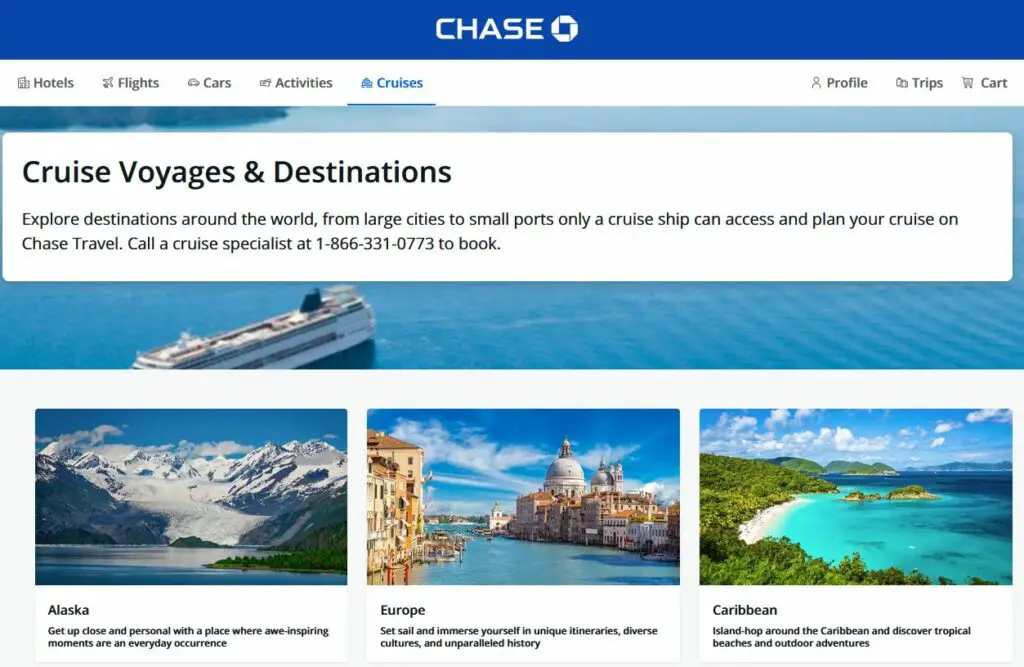This image features a Chase Bank website, specifically from the travel section. At the top of the page, there's a prominent blue bar displaying the word "Chase" alongside the bank's circular logo, which features a white circle with a blue box in the center. The navigation menu includes options such as hotels, flights, cars, activities, and cruises, with "cruises" currently highlighted and underlined. On the right-hand side, there are links to profile, trips, and cart.

In the central section of the page, the heading reads "Cruise Voyages and Destinations." This section invites users to "Explore destinations around the world. From large cities to small ports, only a cruise ship can access and plan your cruise on Chase Travel." A call to action encourages potential travelers to contact a cruise specialist at 1-866-331-07732.

Below this text, there is a vivid image of a stunningly blue sea, part of a pop-up box layered on top of the main content. Further down, three smaller images depict various travel destinations: 

1. Alaska, showcasing majestic snow-capped mountains with a caption inviting travelers to "get up close and personal with a place where awe and inspiring moments are an everyday occurrence."
2. Europe, presenting a beautiful European village nestled by the sea under a clear blue sky.
3. The Caribbean, highlighted by lush green trees, vibrant blue waters, and an inviting sky.

Each image serves to inspire and attract potential travelers, emphasizing the unique and picturesque experiences available through Chase Travel's cruise offerings.